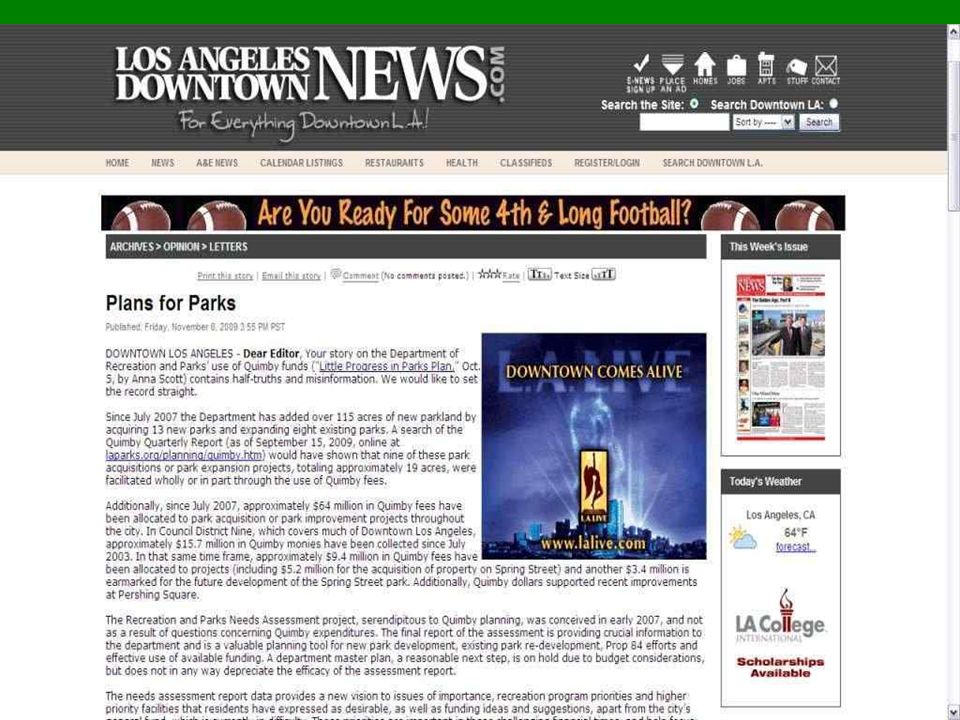This image captures the homepage of the website LosAngelesDowntownNews.com, a comprehensive source for news and events in Downtown Los Angeles. Featured prominently at the top-right section of the page is a search box with the options to 'Search the Site' and 'Search Downtown LA.' The navigation bar underneath includes links to various sections: Home, News, A&E News, Calendar Listings, Restaurants, Health, Classifieds, Register, Login, and an additional search option titled 'Search Downtown LA.' 

Amidst these online functionalities, a banner headline poses, "Are you ready for some fourth and long football?" followed by several sub-sections such as Archives, Opinion, Letters, and Plans for Park. An open letter to Downtown Los Angeles from the Editor critiques an article by Anna Scott published on October 5. The letter claims the story about the Department of Recreational Parks' use of Queen Bee funds and the lack of progress in park plans contains inaccuracies, aiming to correct the record.

Towards the right side of the page, a blue graphic logo catches the eye, portraying a woman at a pool with the text, "Downtown Comes Alive." Below this image, the website URL www.lalive.com is displayed, indicating perhaps an affiliation or highlighting a featured destination within the vibrant Downtown Los Angeles community.